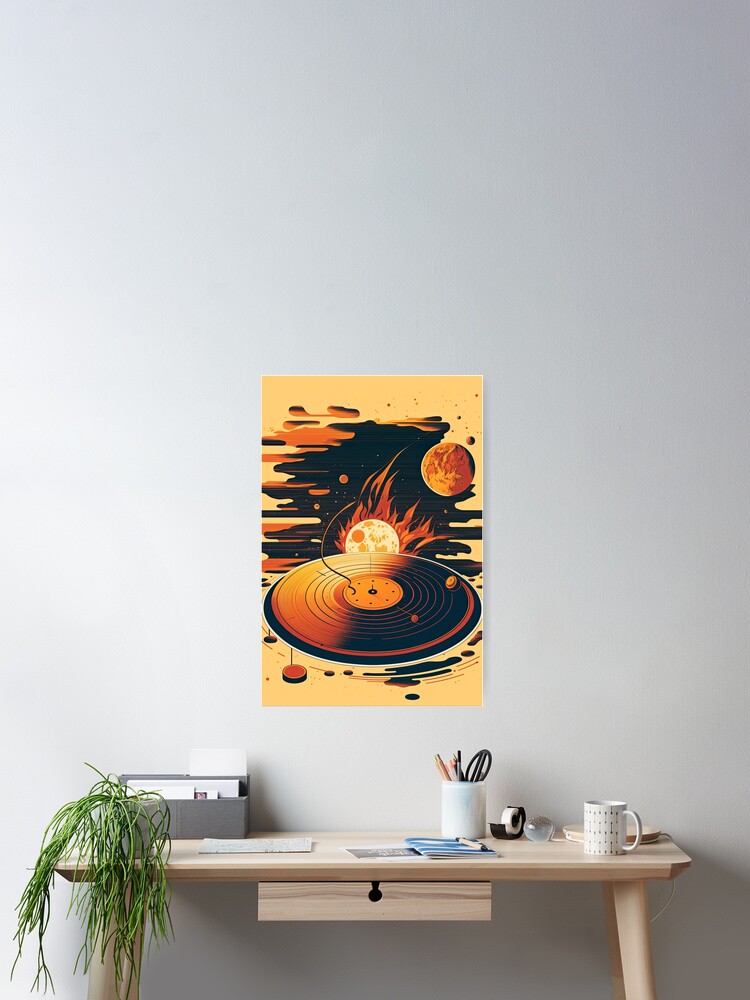The portrait-layout photograph features a corner of a room with a simple light wood desk positioned against a white wall. The desk, centered in the image, stands on four legs and includes a small drawer in the middle with a keyhole. On the desk surface, there is an assortment of items: a small white lamp to the right, a white mug, a white cup filled with pencils and scissors, a roll of tape, a little green houseplant, and a grey letter sorting holder containing various papers and booklets. 

Mounted above the desk is a portrait-layout painting with a creamish-yellow background, depicting a record player spinning a disc. The artwork includes elements of black, orange, and red hues, creating a vibrant scene. Two planets, one appearing fiery, float in the black and orange-splattered cosmos behind the record player. This painting adds an intriguing and artistic touch to the entire setup, blending the themes of music and space seamlessly into the room's decor.